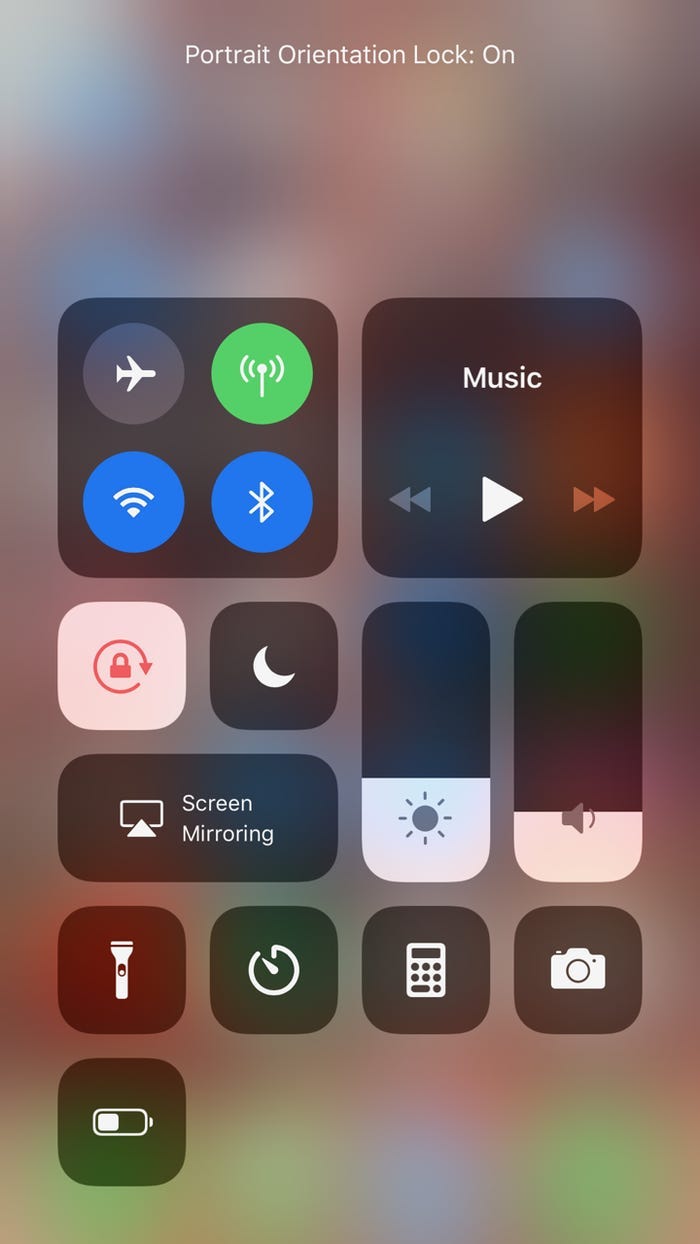This image captures a detailed view of a smartphone control center screen. The background is a grayish-blue hue. 

At the top, the "Portrait Orientation Lock" is highlighted, indicating that the screen orientation is locked in portrait mode. Directly beneath this, there's a grid of square icons. The first icon features an airplane within a circle, signifying Airplane Mode. Next, a green circle icon represents Wi-Fi, adjacent to which is a blue circle showing the current Wi-Fi connection status. Beside this is another blue circle, signifying Bluetooth.

Further down, a black square labeled "Music" displays media control icons, including a play arrow, a back arrow, and a skip ahead arrow. Beyond the music controls, there are more functional icons: one to lock the screen, another for nighttime mode, screen mirroring, audio controls, and screen brightness adjustment. There's also a flashlight icon and a semicircular arrow pointing left, the function of which is not immediately clear. The bottom row includes icons for the calculator, camera, and a battery level indicator.

This detailed depiction of the smartphone control center provides quick access to various settings and media controls.